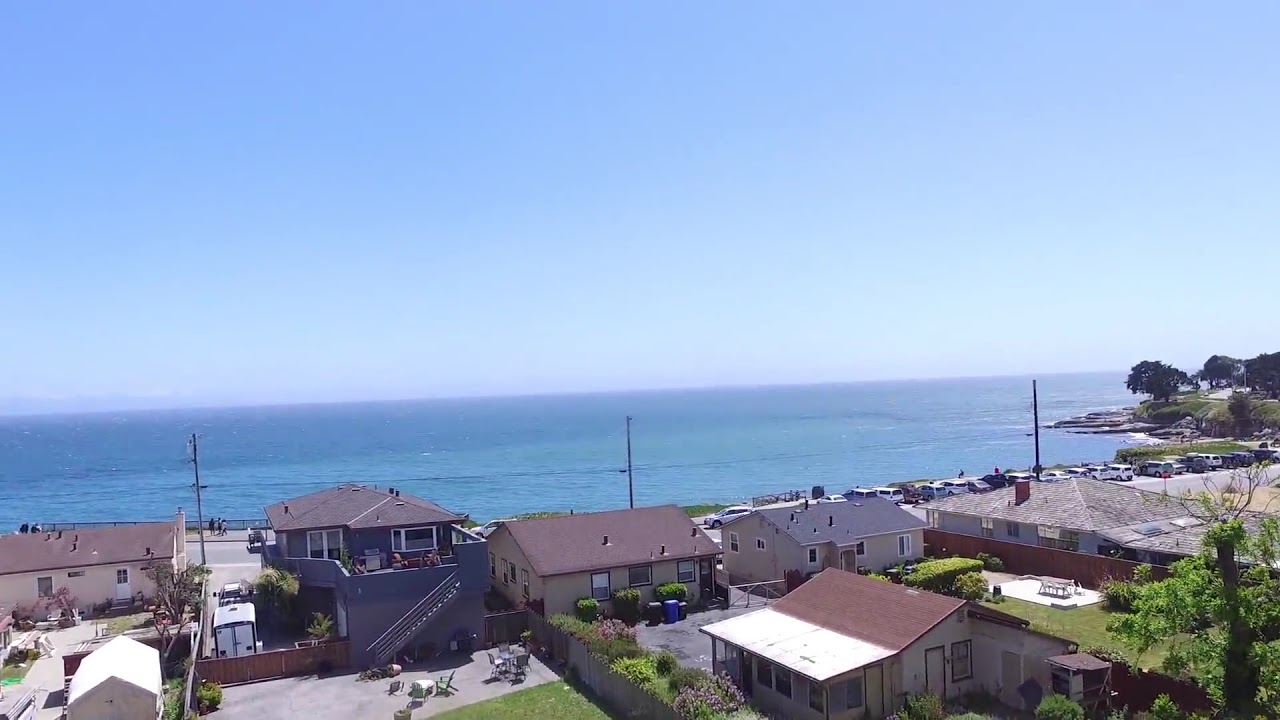This aerial color photograph in landscape orientation captures a picturesque coastal village nestled by the expansive, shimmering ocean. The residential area in the foreground features five to six houses of varying heights, some reaching up to three stories. Dominating the center is a gray house with a set of gray handrailed stairs, alongside two patio chairs that appear to have been toppled by the wind. Near this house stands a table with four upright chairs. Moving to the right, there is another house with a red tile roof and next to it a smaller beige house with a light gray roof. Further right lies a larger house that stretches from the ocean towards the edge of the image. A prominent two-story house with a white staircase and another beige house are positioned on the left.

The village extends from the right side to the left side towards the foreground, framed by a clear blue sky that occupies the top 60% of the image. The ocean transitions from a dark blue hue at the horizon to lighter blue near the shore, where an island outcropping juts out. Scattered trees and telephone poles accentuate the shoreline, and a parking area is visible with cars parked beyond the buildings and slightly to the right. The serene aerial view emphasizes the harmonious coexistence of human habitation and natural beauty, captured perfectly through drone photography.